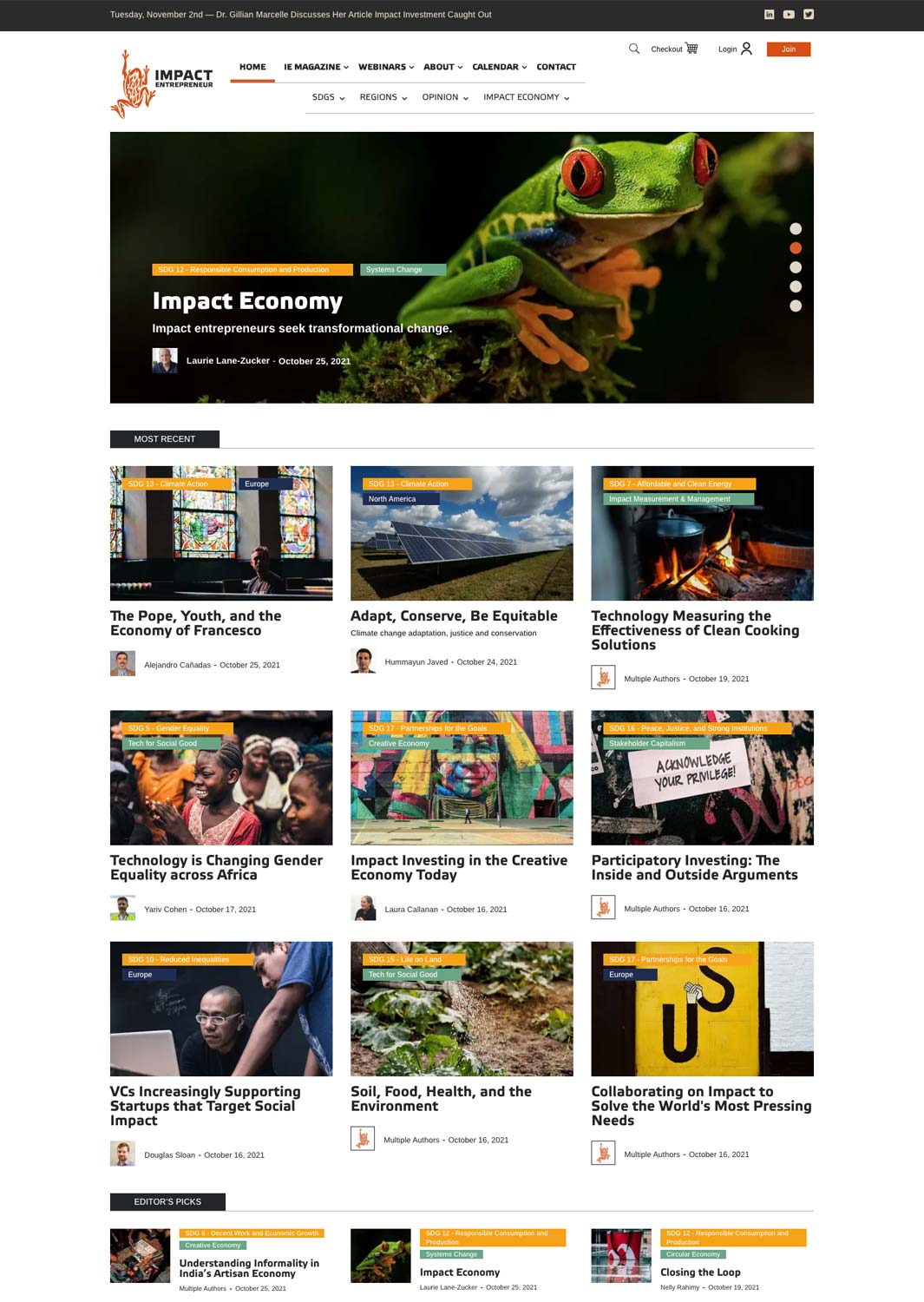The homepage of Impact Economy is displayed prominently with a distinctive logo that resembles a frog and the text "Impact Economy" in bold black letters. The navigation bar is present but the details are not legible. A highlighted article titled "The Pope, Youth, and the Economy of Francesco" is featured, signaling that the site focuses on economy-related content. Beneath this main article, there are eight to nine tiles showcasing various other articles, all under a section labeled "Popular." The splash screen, dominated by the Impact Economy frog logo, is part of a five-image carousel, currently on the second image as indicated by the highlighted second dot out of five dots at the bottom. In the top right corner, there is a small login field, which is difficult to read due to its size.